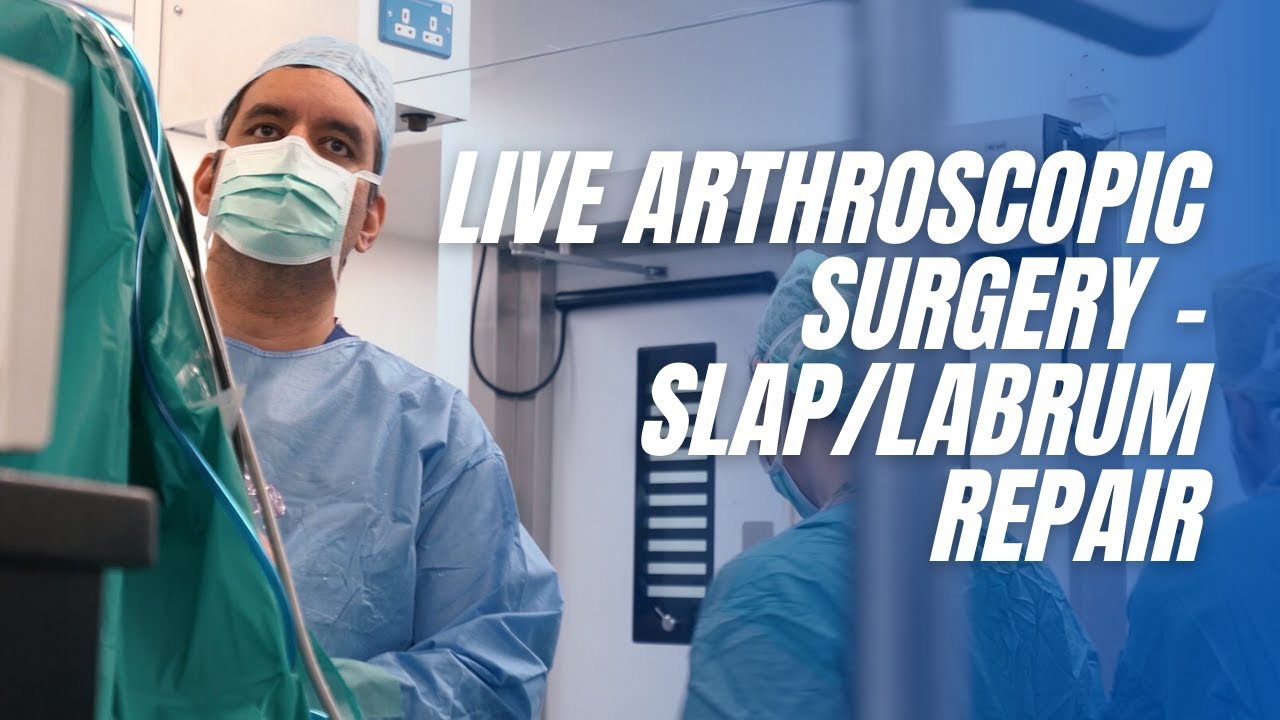The image is an advertisement featuring prominent white letters stating "LIVE ARTHROSCOPIC SURGERY – SLAP/LABRUM REPAIR." On the right side, the back of a surgeon or nurse in blue scrubs is visible. In contrast, the left side shows another healthcare professional in blue scrubs and a mask, looking towards the viewer. Blue-green surgical equipment can be seen on the left edge. Between the two professionals is a doorway, with the background consisting of the white interior of a medical building, indicating a clinical setting where preparations for surgery are underway.